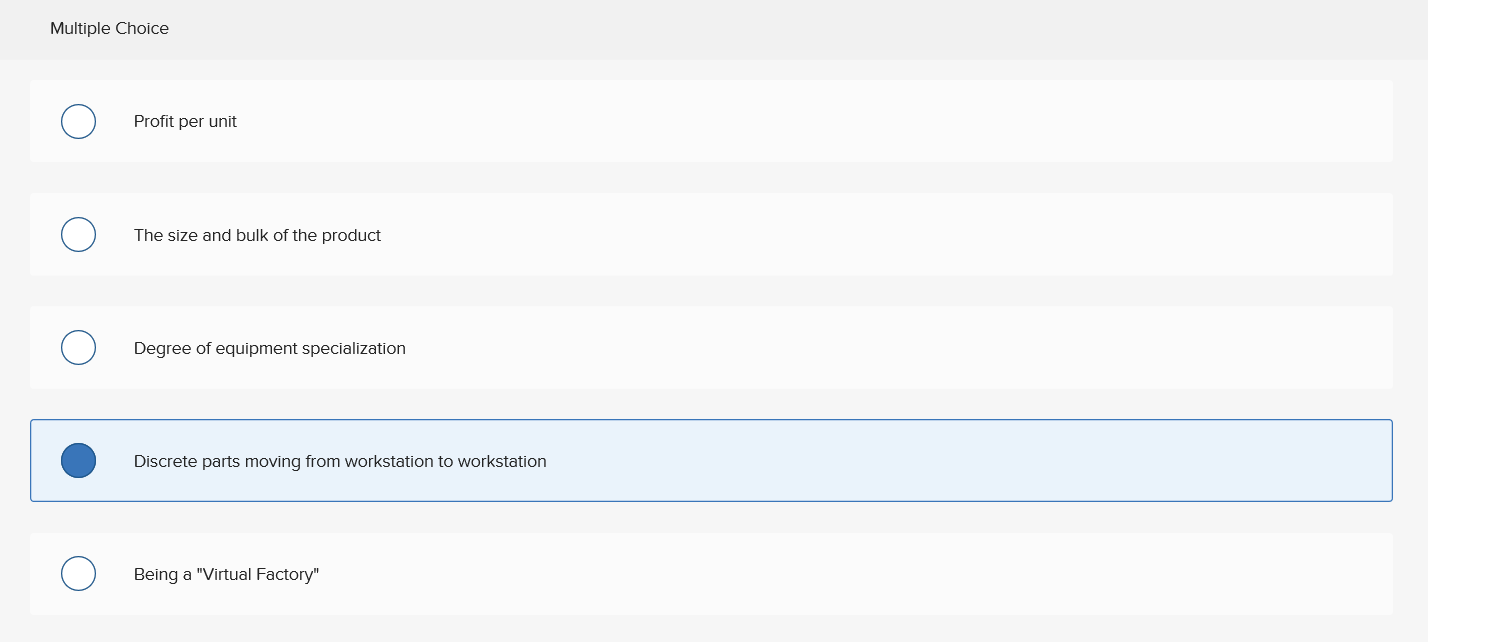The image depicts a multiple-choice test question displayed on a gray background. The title at the top clearly states "Multiple Choice" in black text. Below this title, there is a single multiple-choice question with five different answer options:

1. **Profit per unit** 
   - Next to this option on the left is a small, unfilled circle.
2. **Size and bulk of the product**
   - This option also features an unfilled circle to its left.
3. **Degree of equipment specialization**
   - An unfilled circle is positioned to the left of this option as well.
4. **Discrete parts moving from workstation to workstation**
   - This option is highlighted with a blue box, and the circle to its left is filled in blue, indicating it as the selected answer.
5. **Being a "virtual factory"**
   - An unfilled circle is located to the left of this option.

All text for the question and options is in black. Each option is enclosed within a light gray or white box that spans from the left of the circle to the right edge of the page. The chosen answer, "Discrete parts moving from workstation to workstation," is distinctly highlighted in blue for emphasis.